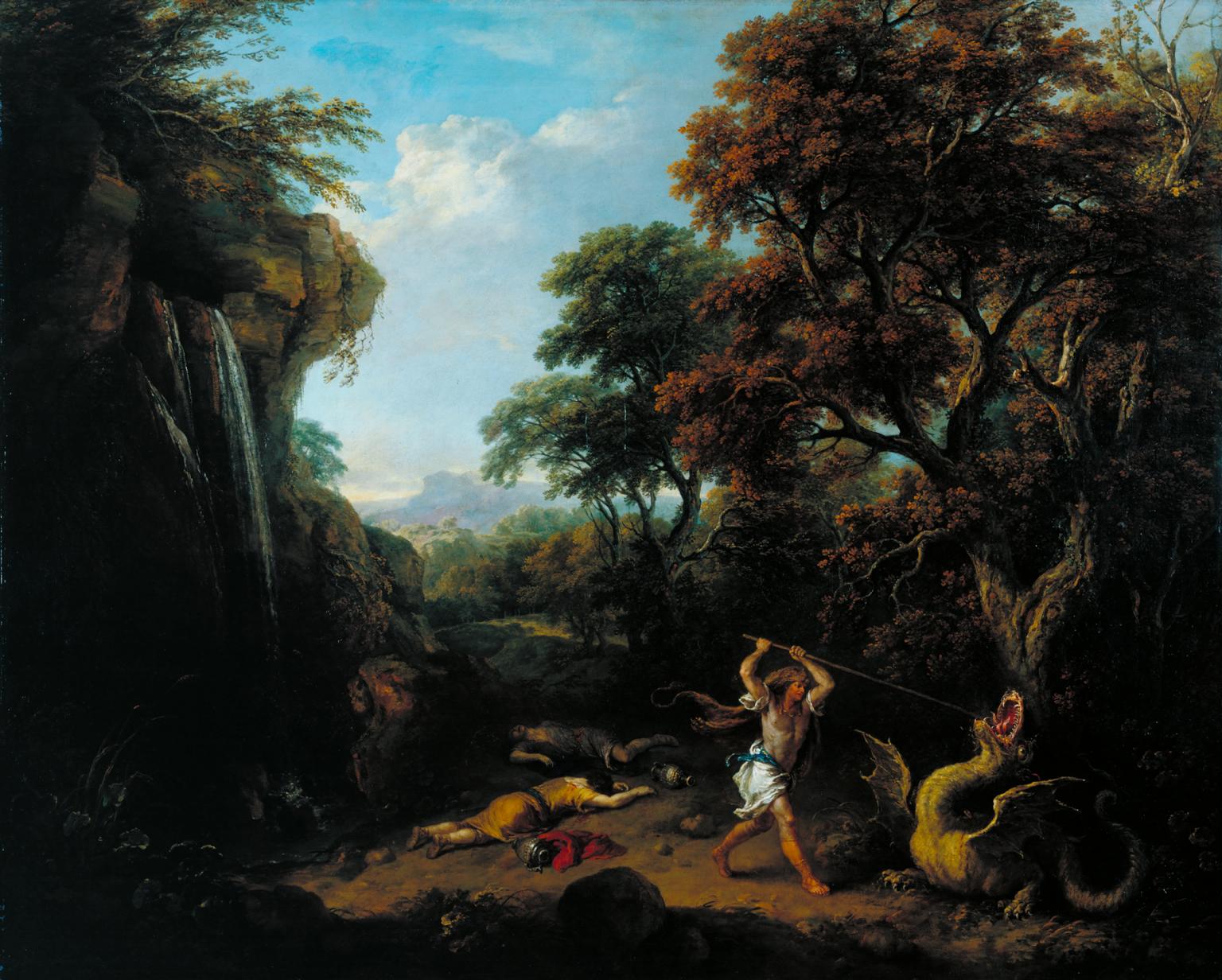The painting depicts a dramatic and gruesome scene of a young, muscular warrior, possibly a woman, engaged in a fierce battle with a dragon. Clad in a loincloth, the warrior is seen thrusting a long metal pole or a spear into the dragon's throat, which writhes in agony. The dragon is of similar size to the warrior, with wings and a long tail. Lying on the blood-soaked ground around the combatants are several dead or distressed individuals, perhaps victims of the dragon's earlier wrath, some of whom were carrying jugs that might have contained wine. Behind them, the forest is dark and twisted, with gnarled and knotty limbs, and brown, lifeless foliage. This foreground scene starkly contrasts with the background, where verdant green trees, a blue sky filled with many clouds, and distant mountains provide a glimmer of serenity. A waterfall cascades down to the left, adding a touch of motion to the stillness of the tragic tableau. This image, which could be a print of a painting from an era reminiscent of Michelangelo or Raphael, captures a moment of mythological or fairytale intensity.